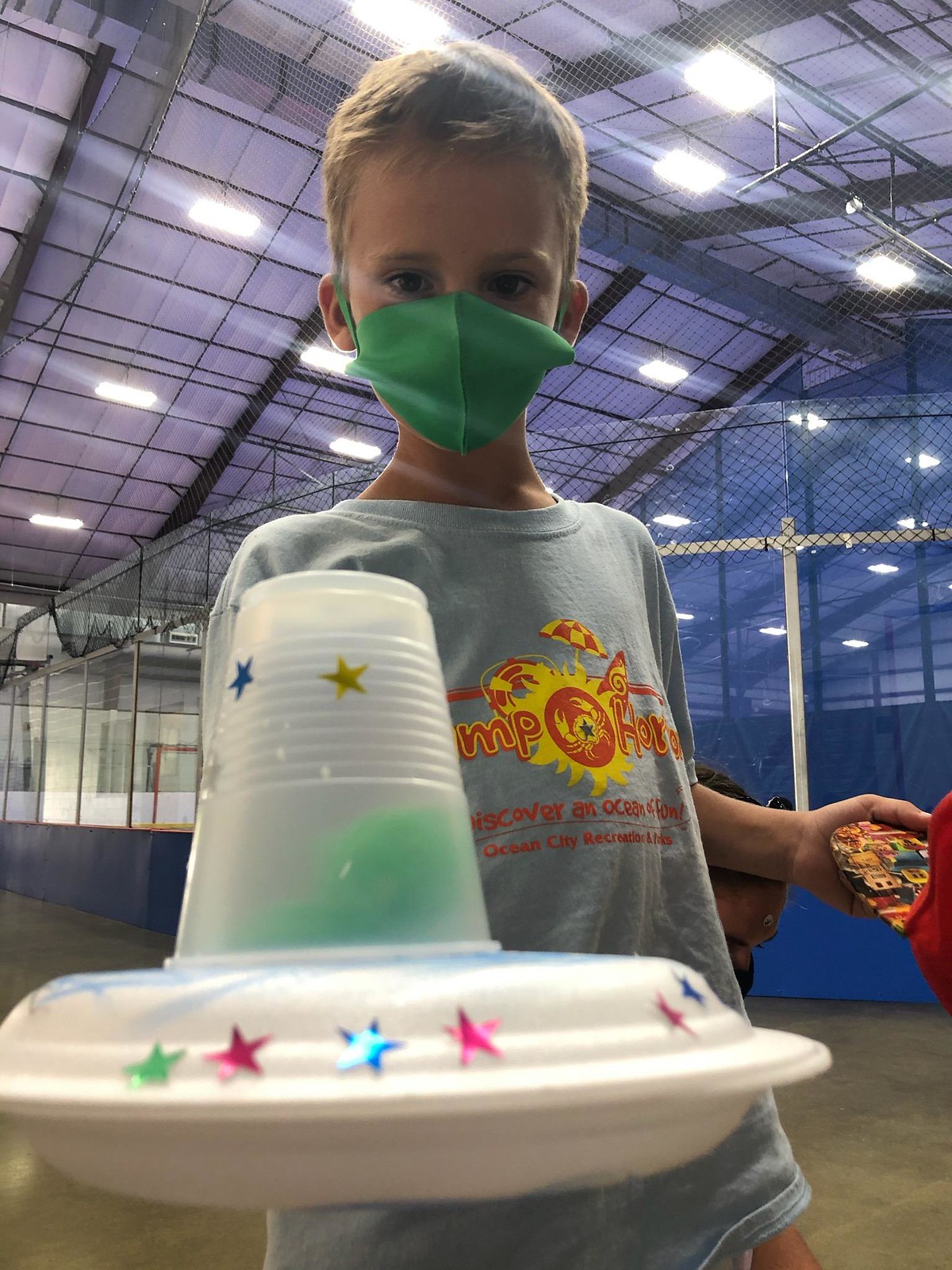The image features a young Caucasian boy, around eight to ten years old, standing in an indoor setting with high roofs and fenced walls, possibly a large building or summer camp. The boy takes up most of the frame. He has blonde to light brown hair and is wearing a green protective mask typically used for health reasons. His outfit consists of a gray shirt with red and yellow text, depicting a crab, sun, and beach umbrella.

In his right hand, the boy is holding an intricate craft: two styrofoam plates stacked opposite each other to form a UFO-like compartment, adorned with glittery star stickers in blue and yellow. Additionally, an overturned plastic cup, also covered in star stickers, sits atop the plates. In his other hand, he appears to be holding a hat. Behind him, there is a partially visible woman who is also wearing a mask.